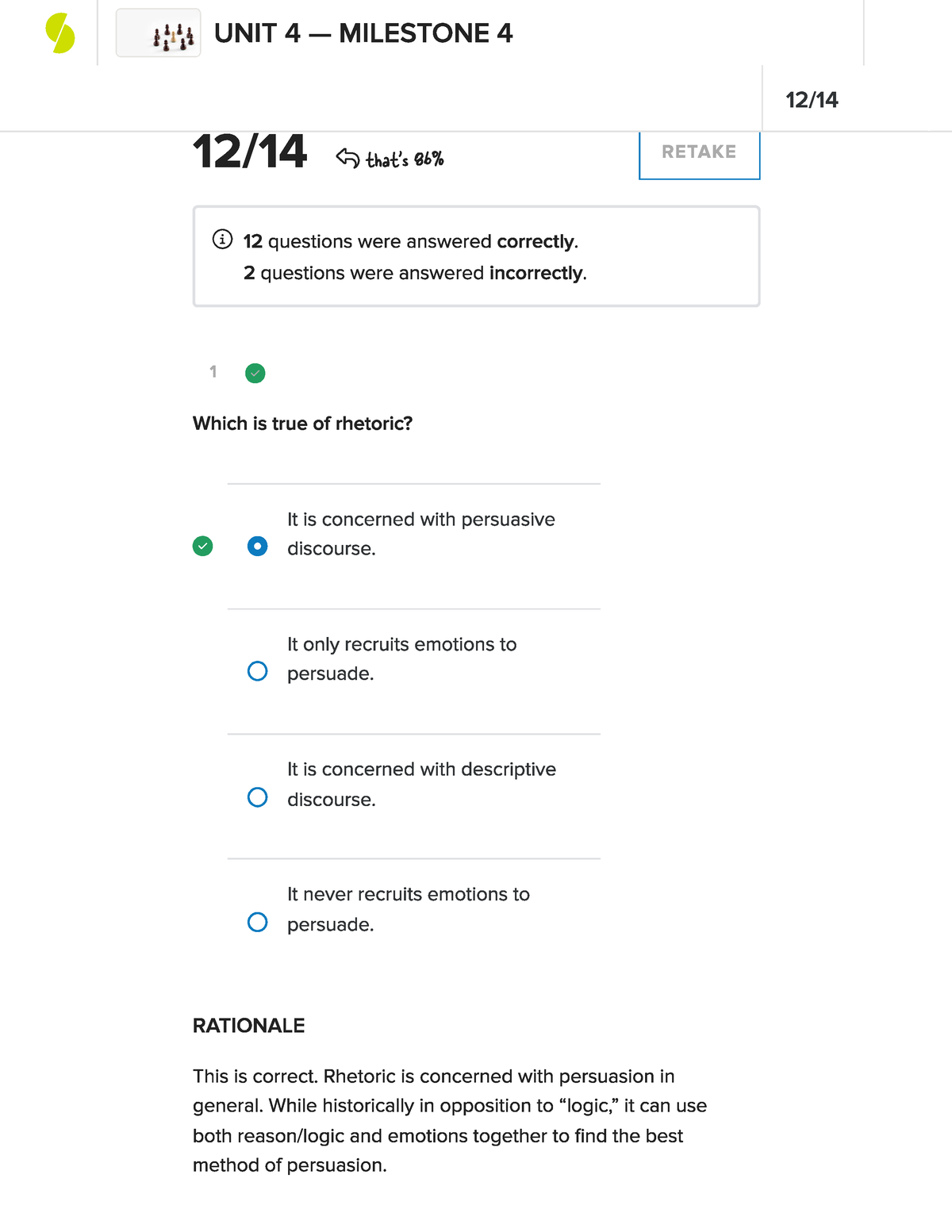This image displays a screen labeled "Unit 4 Milestone" and "Milestone 4." To the right of this label, there is an icon featuring two halves of a green circle, tilted slightly. 

The upper left corner of the image shows the date "12/14" with another instance of "12/14" directly below it, accompanied by a small arrow pointing to the second date. Next to this arrow, the text "86%" is displayed, indicating a score. The score notation appears somewhat casual and is distinct from the rest of the text, which is in a more standard font size of 14. To the right of this section, there is a button labeled "Retake."

Beneath this, a box contains additional information: it states that "12 questions were answered correctly" and "2 questions were answered incorrectly." The image also includes a sample question about rhetoric with multiple-choice answers. The correct answer has been selected and is marked with a filled circle and an arrow pointing to it. The correct answer is "It is concerned with persuasive discourse."